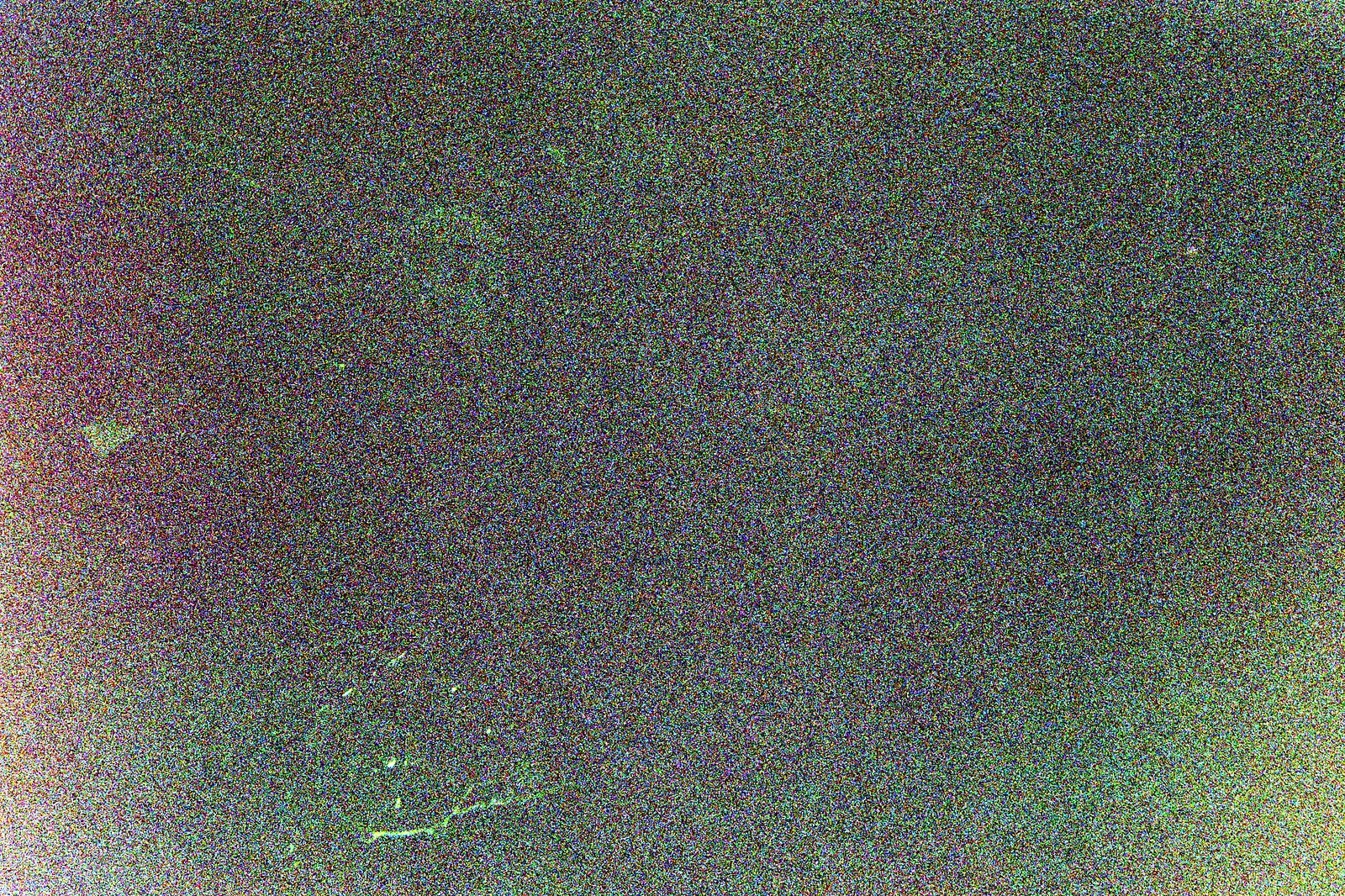The image is a highly pixelated and grainy photograph in landscape format, reminiscent of a television screen displaying static noise or an out-of-signal image. The composition is predominantly composed of very dark, almost black dots interspersed with greenish light blue and dark purple spots. Accentuating the lower right corner, a yellowish tint hints at light emanating from this area. If the image were to be divided into thirds, a notable white line resembling a spit trail appears slightly to the left of the bottom center, accompanied by a white spot to its left and a more dense concentration of purple dots behind it. The left side of the image ambiguously features shapes that could be interpreted as a face with black eyes and eyebrows, and possibly a foot outlined in white and green. The upper part of the image, as well as patches scattered throughout, exhibits a blend of green, red, and black colors, contributing to the overall multicolored and abstract quality of the photograph.